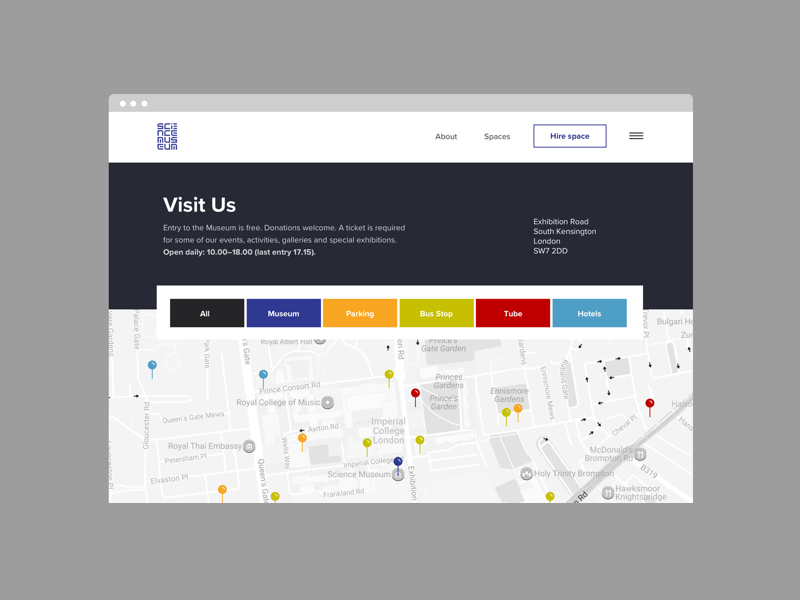This is a detailed screenshot of a website with a central pop-up window, framed by a thick gray border. The title "Science Museum" is displayed at the top left in a somewhat hard-to-read format as each word is split into three-letter rows. To the right, the top of the screen lists navigation options: "About," "Spaces," and "Higher Space," the latter highlighted in a purplish-blue rectangle. 

Below this navigation bar, the website features a dark blackish background with the following text: 

- **Visit Us**
  - Entry to the museum is free; donations welcome.
  - A ticket is required for some events, activities, galleries, and special exhibitions.
  - Open daily 10:00 - 18:00, last entry at 17:15.
  - Location: Exhibition Road, South Kensington, London, SW7 2DD.

Underneath this information, there are clickable options labeled "All," "Museum," "Parking," "Bus Stop," "Tube," and "Hotels." A gray map displaying the surrounding area is positioned below these options, with color-coordinated pinpoints corresponding to each category, such as red pins indicating tube stations.